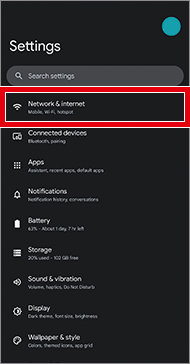In the top-level settings hierarchy interface in night mode, the image prominently features a green circle in the upper right corner where typically the Google account avatar resides. This user has either not set an avatar or opted for a simple green circle. Directly below this, the heading "Settings" is clearly visible, followed by a search box adorned with a magnifying glass icon, prompting users to "Search settings." A bold red rectangle, likely added through post-processing, highlights the first subheading in the settings list, "Network and Internet." The background of the interface is black, making the white text stand out sharply. Other visible subheadings in the settings hierarchy include "Connected Devices," "Apps," "Notifications," "Battery," "Storage," "Sound and Vibration," "Display," and "Wallpaper and Style."